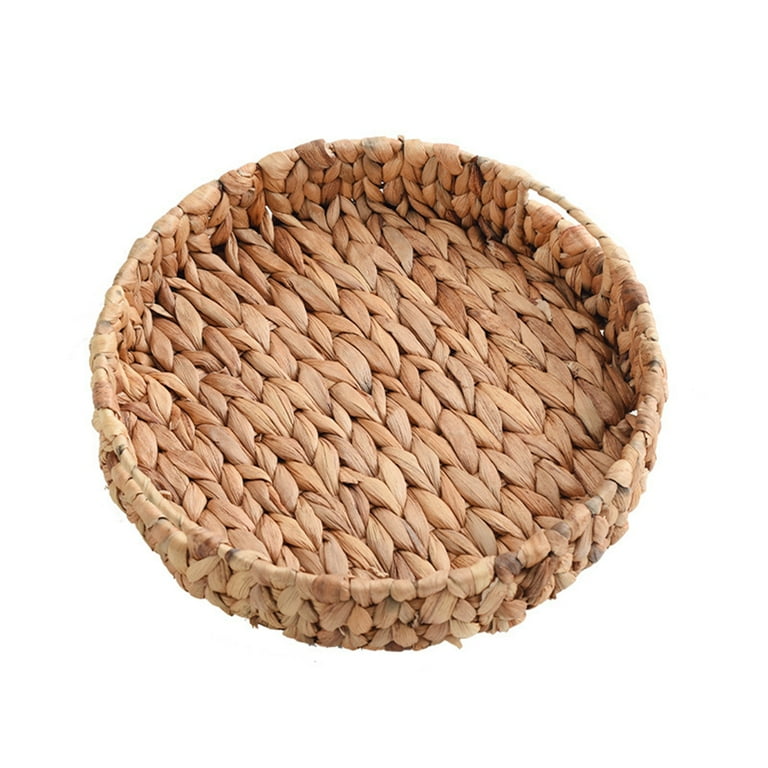The image shows a circular, woven tray that appears to be made from raffia or wicker, exhibiting various shades of beige and darker browns. The weave creates small bulb-like formations resembling cloves of garlic. The tray is shallow, suggesting it could hold small items like television remotes, magazines, drinkware, or coasters. It features two thin handles, one on each side, giving it a delicate, functional aspect. Photographed from a top-down perspective at a slight angle, the background is a plain white, making the tray appear as though it is floating. The craftsmanship is intricate, with the braid neatly wrapped around a basket-like frame, creating an overall beautiful and delicate appearance.